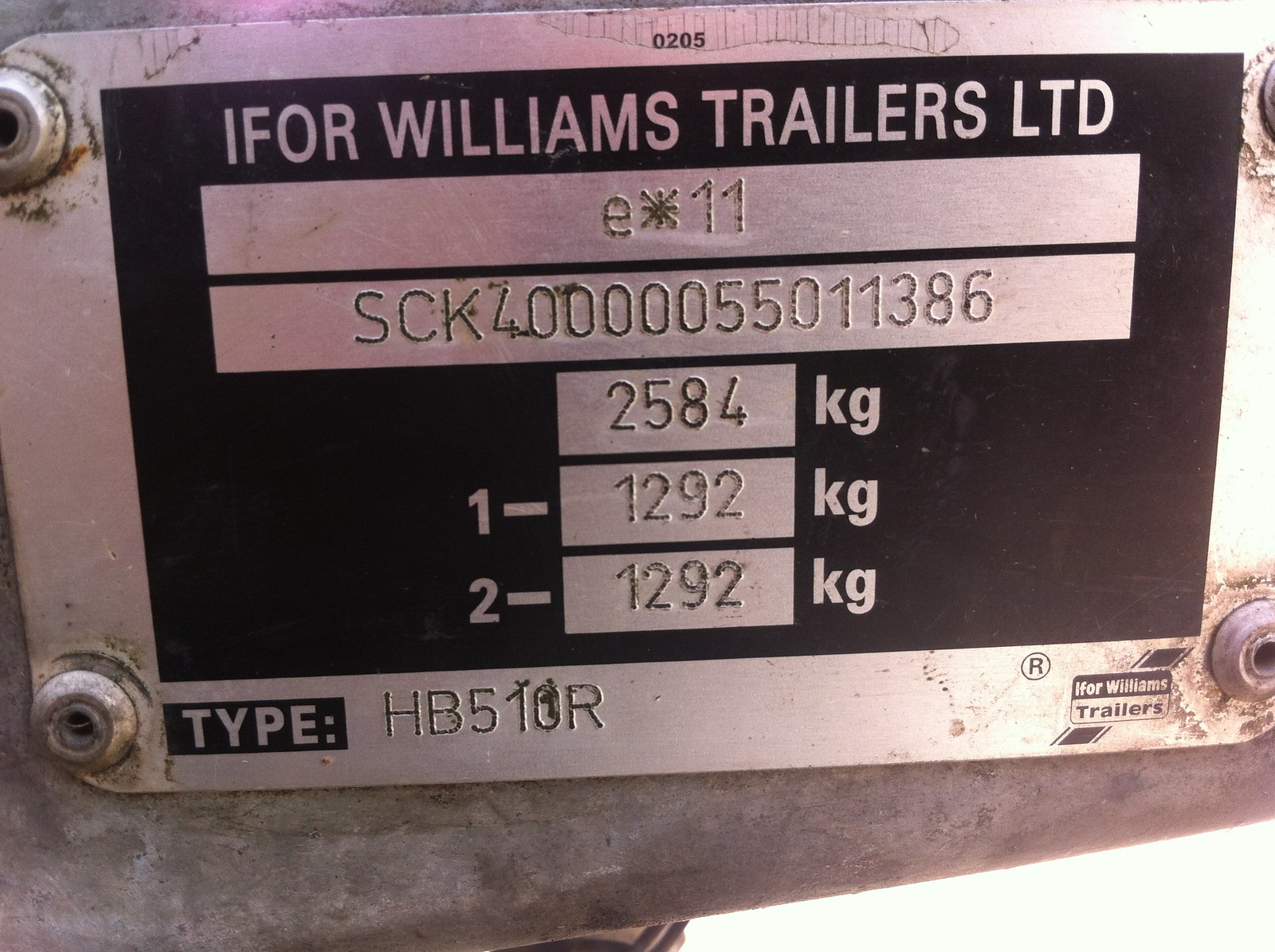This is a detailed close-up photograph of a metal plaque that appears to belong to a trailer from IFOR Williams Trailers Ltd. The plaque itself is held in place by bolts and mounted on a metal platform. The plaque features a prominent black background with silver and white text. At the top of the plaque, the inscription reads "0205 IFOR Williams Trailers LTD." Directly beneath this, in a rectangular box, it says "e*11."

Further down, another rectangular box contains a serial or identification number: "S-CK-400000-55011-386." Below this are three smaller boxes displaying weight information: the first box reads "2584-KG," the second box with a "1-" prefixed reads "1292-KG," and the third box with a "2-" prefixed reads "1292-KG."

At the bottom left of the plaque, the word "TYPE" is engraved, followed by "HB510R." The branding "IFOR Williams Trailers" appears again at the bottom right in smaller lettering. The overall image captures the plaque clearly, emphasizing the detailed inscriptions and the metallic finish against the contrasting background.